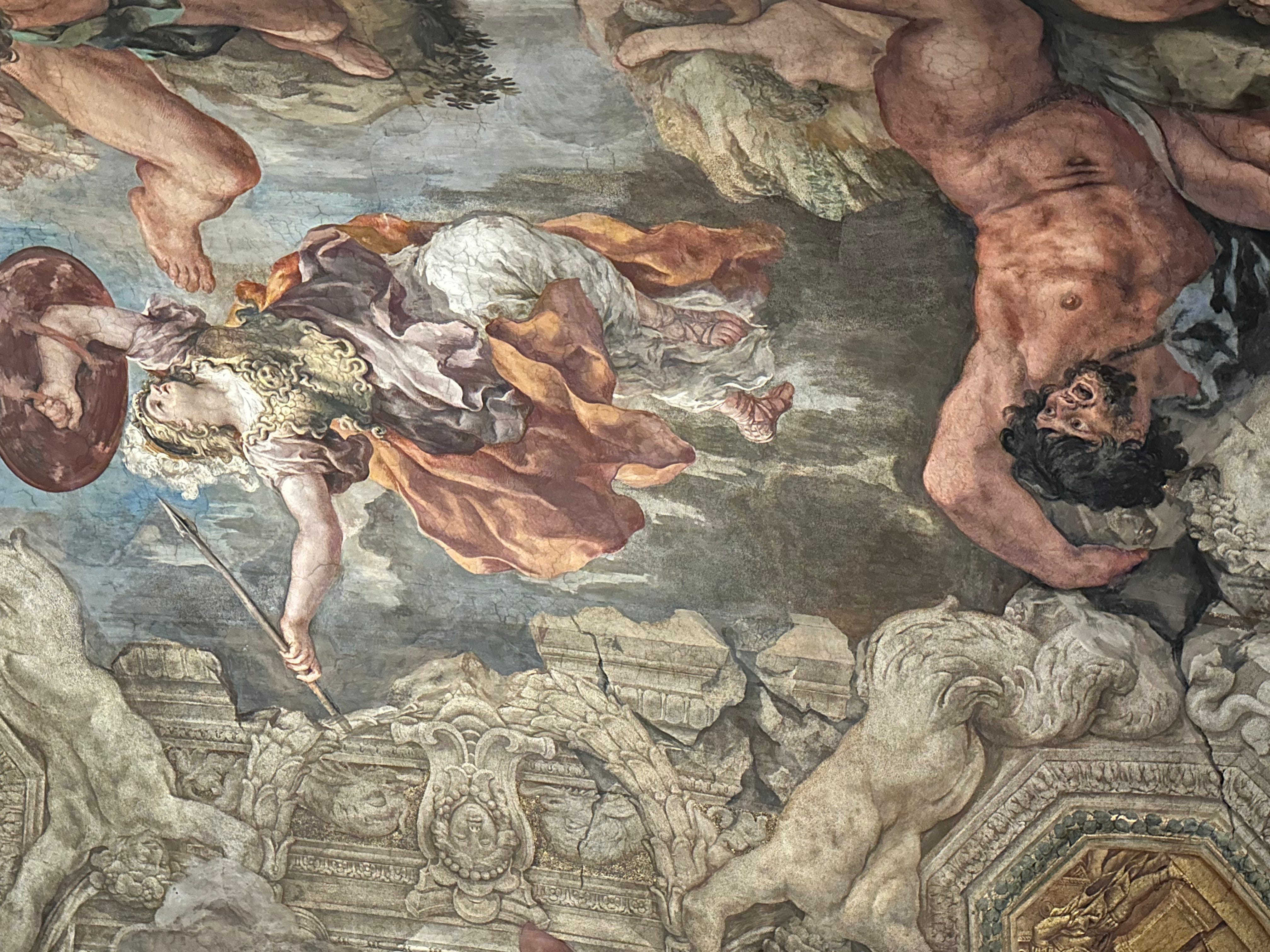This detailed artwork from the Sistine Chapel, painted by Michelangelo, showcases an intricate blend of vibrant and classical elements. Dominating the scene is a partially nude man with dark hair and a beard, positioned upside down on the right side with a perplexing expression. To the left, a woman is depicted sideways, draped in flowing gold, purple, and white fabric. She wields a spear and shield, embodying a striking classical figure. Both figures are surrounded by three-dimensional moldings and cherubs, with some appearing to have serpentine tails. The background reveals the rock and plaster peeking through, suggesting the passage of time and the enduring nature of the masterpiece.